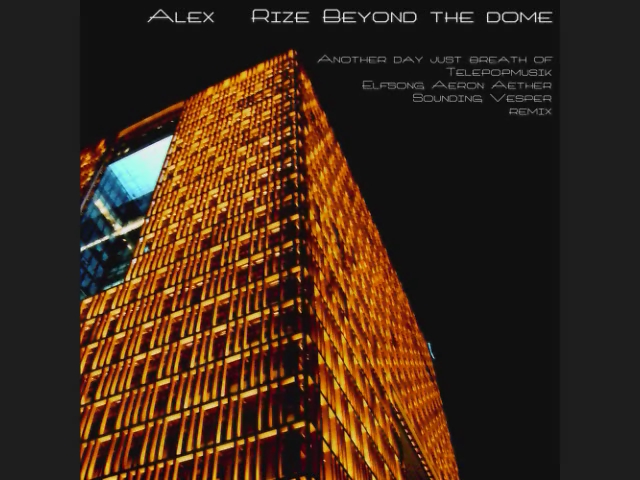The image appears to be a poster or album cover set against a dark, almost black background. Dominating the composition, slightly off-center to the left, is a tall building glowing in a golden, amber hue with some black accents. The perspective is from below, looking upward towards the structure that features one prominent window near the top. The text, in white, occupies the upper portion of the image and reads, "Alex, rise beyond the dome." Below this headline, a list of names and phrases is stacked vertically: "Another Day, Just Breath, Telepop Music, Elf Song, Aaron Ather, Sounding Vesper," concluding with the word "Remix." The limited color palette includes shades of black, dark grey, various tones of gold, and white, enhancing the striking visual impact of the illuminated building against the dark background.